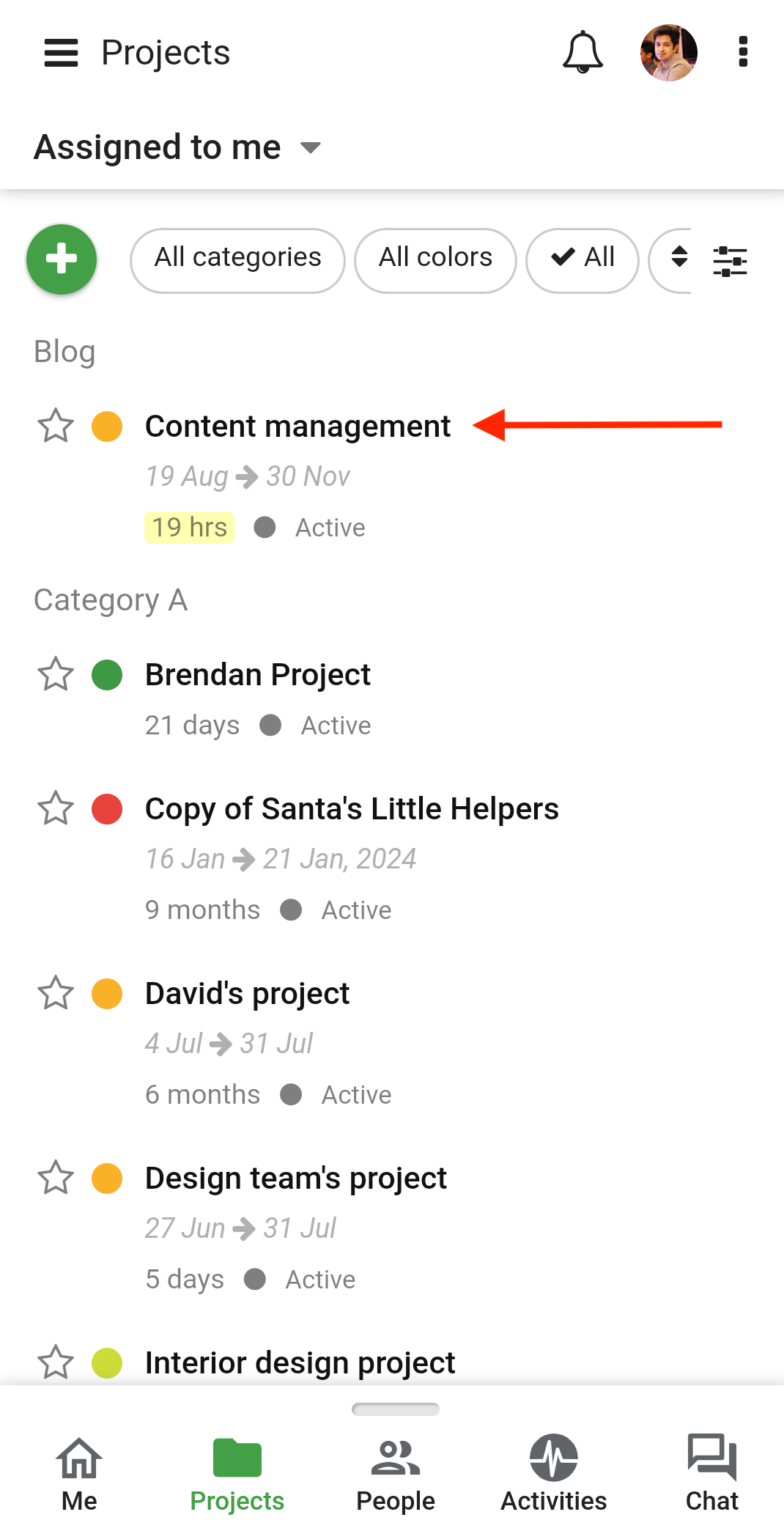**Detailed Description for the Image Caption:**

The image is a screenshot from a cell phone displaying a project management application interface. At the top, there is a header labeled "Projects," accompanied on the left by an icon with three horizontal lines stacked vertically. Beneath the header, along the left margin, a menu item labeled "Assigned to Me" features a downward-pointing arrow.

Toward the top left corner, a white plus sign within a green circle is prominently displayed. To the right of the plus sign, there are various filter options, including "All Categories," "All Colors," and an "All" checkbox.

Under the plus sign, a list of project categories is shown. The first item, marked with a star and a yellow circle, is labeled "Content Management." This project spans from August 30th to November 30th, with a total of 19 hours allocated to it and a status indicator marked "Active." A red arrow digitally points to this specific project.

Further down, the list continues with categories and associated projects, each tagged with a colored circle:
- "Category A" with a green circle labeled "Brendan Project."
- A red circle labeled "Copy of Santa's Little Helpers."
- An orange circle for "David's Project."
- Another orange circle for "Design Team's Project."
- A green circle for "Interior Design Project."

The interface is neatly organized, making it easy to identify and navigate through different projects and their details.